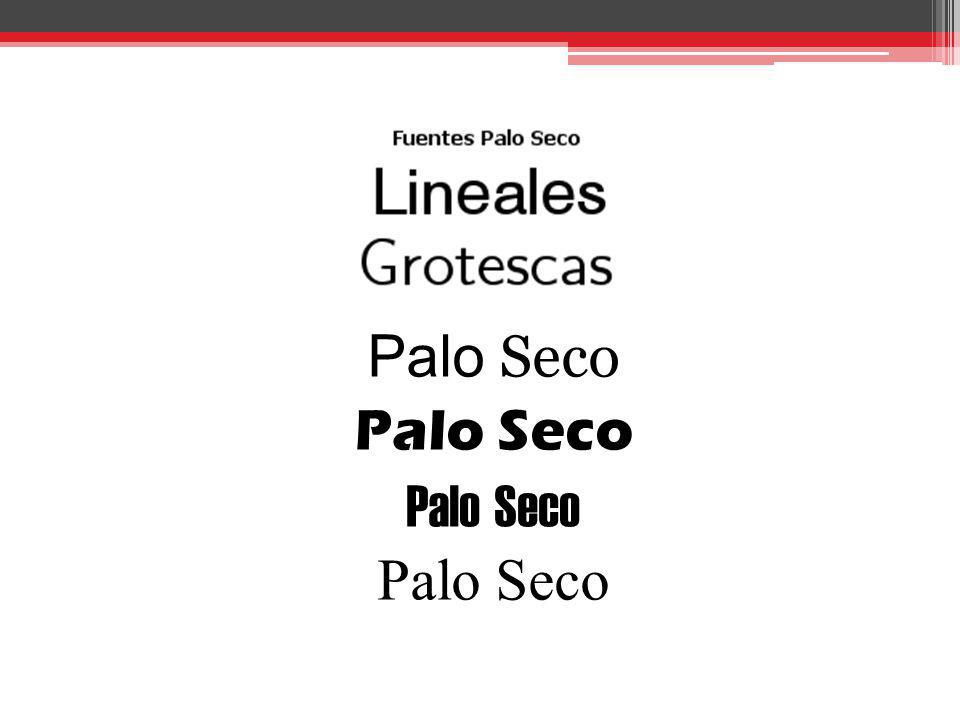The image features a white background upon which various fonts are showcased. At the very top, there is a gray color block that fades into white via a harsh gradient. Below this block are a series of horizontal lines, including red lines and a thin pink line, also fading into the gradient. Centrally aligned on the page are lines of text in black, each line featuring words like "Fuentes," "Palo Seco," "Lineales," and "Grotescas." These words are presented in different font styles and weights, with some fonts being bold, others thin, and various sizes, ranging from smaller to larger text. The sequence of "Palo Seco" is repeated several times, each instance in a distinct font. All the text is written using both uppercase and lowercase letters, making the visual arrangement appear like a typographic display or a slide from a presentation.